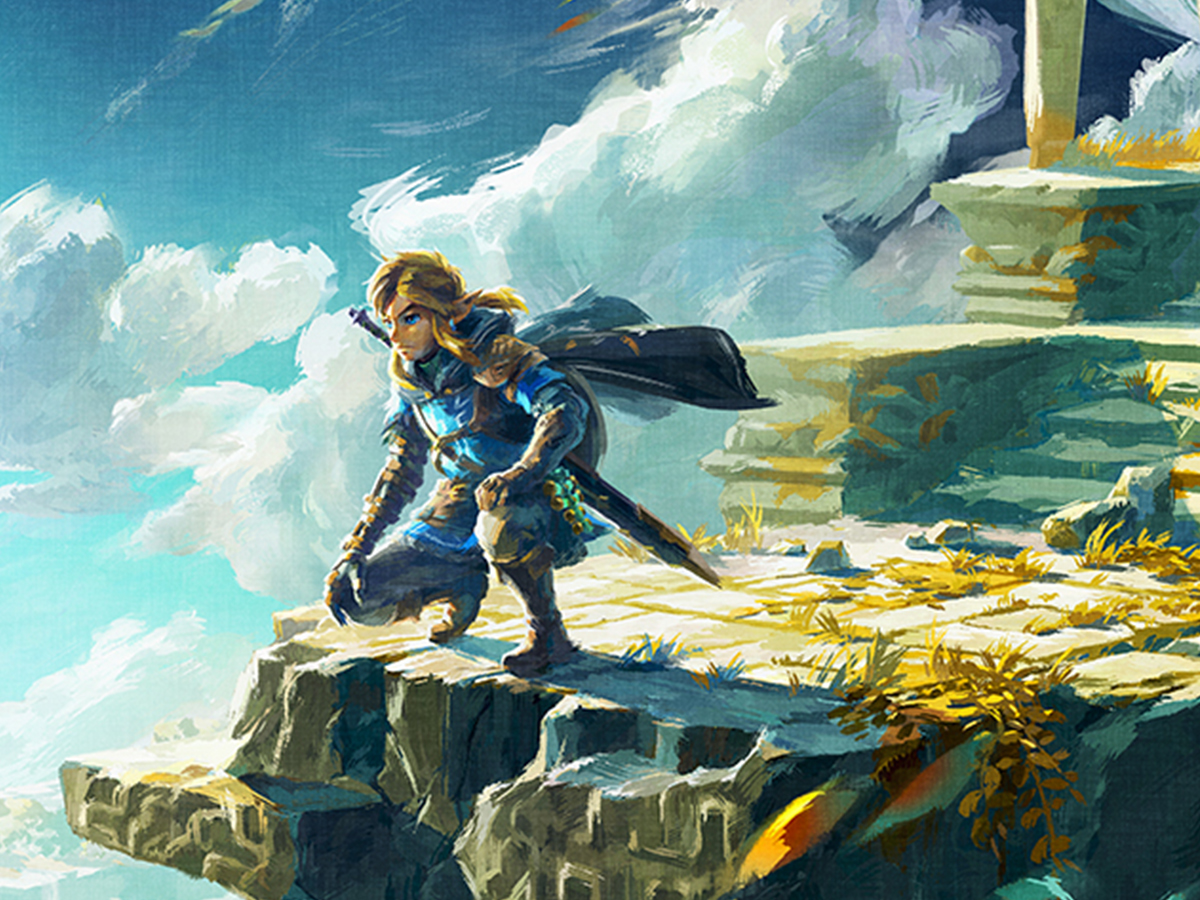This is a detailed painting that vividly captures an elvish-like warrior figure kneeling on a broken cliff or man-made ruin with a dramatic backdrop. The warrior, who may be male, has distinct pointed ears, a pointed elvish face, and is dressed in glimmering blue armor with gold accents. Long, flowing hair cascades down, blending with the matching blue cape that billows dramatically in the wind behind them.

The figure wears high-top black boots, and their knees hover just above the ground in a crouched position, showcasing a fierce, determined expression on their face as they glance to the left. A long dagger or sword is strapped diagonally across their back, adding to their warrior-like appearance.

The setting is a large, collapsed stone precipice with visible layers and stairs leading up to the right. Goldenrod hues and teal tones are interspersed among the stone, with yellow weeds and perhaps foliage hinting at an ancient, crumbling structure. A broken railing and a column stand nearby, adding to the sense of an old, forgotten place.

Above, a blue sky adorned with puffy, swirling clouds fills the upper left corner, gradually becoming more prominent towards the middle. The entire scene is painted in muted tones of blue, gray, and gold, contributing to the epic and slightly melancholic atmosphere of the artwork.